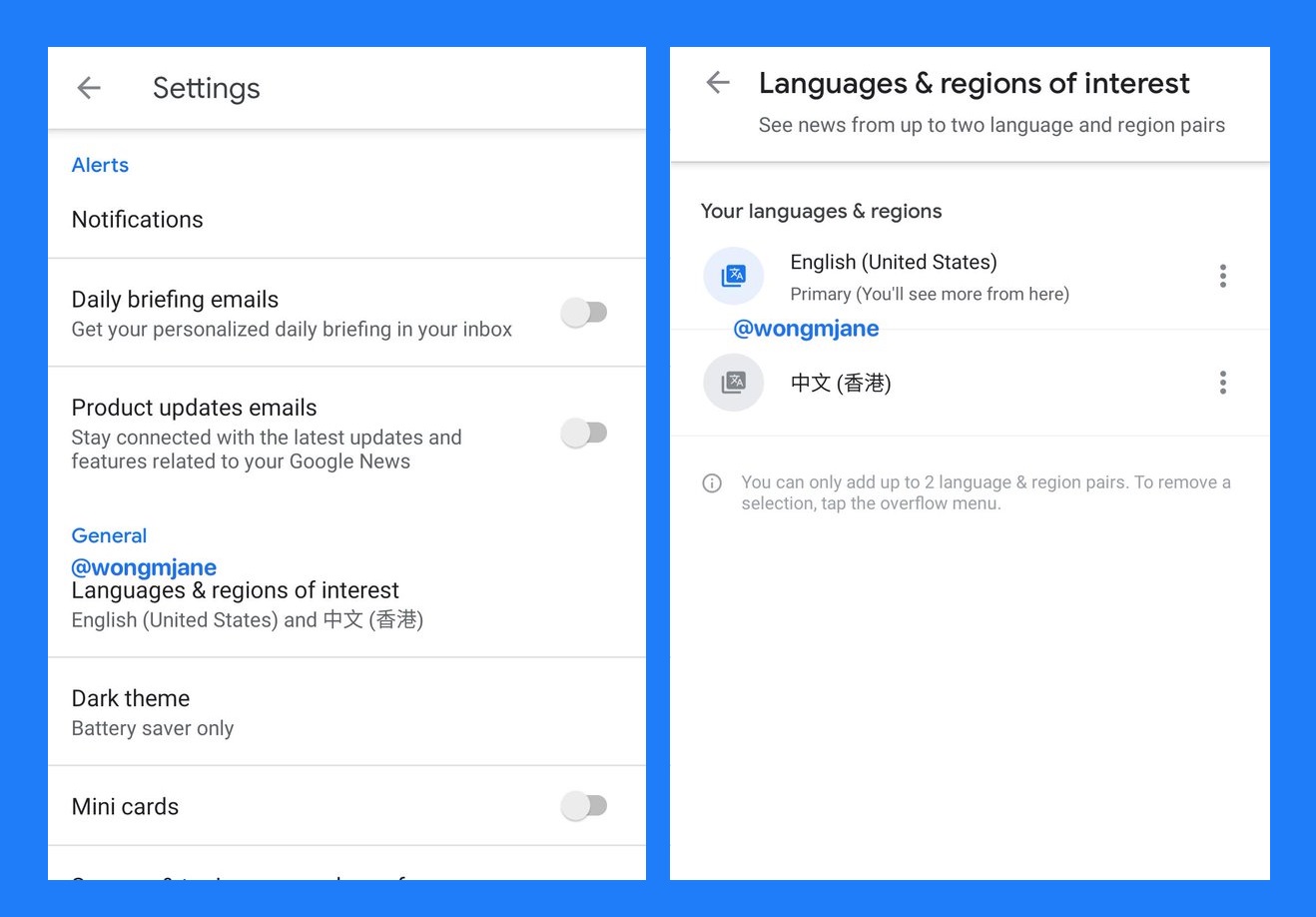Two screenshots with a teal blue border encompassing them are displayed side-by-side, divided by a line running vertically down the center. Both screenshots feature a white background and a gray left-arrow icon on the left side. 

In the left screenshot, the title "Settings" is displayed at the top, with blue categories listed below: "Alerts," "General," and "Wong M. Jane." These categories are written in black font, with some options accompanied by sliding toggle bars.

The right screenshot is titled "Languages and Regions" in bold black font. Beneath this, in lighter gray text, it reads "Select up to two languages and region pairs." There is a section titled "Your Languages and Regions," where "English" is selected, and "Wong M. Jane" appears in blue. Additionally, there is another language, presumably Chinese, represented by unreadable symbols. Further down, in gray text accompanied by an eye icon within a circle, it states, "You can only add up to two languages and region pairs. To remove a selection, tap the overflow menu."

The layout is very simple and symmetrical, enhancing its readability.